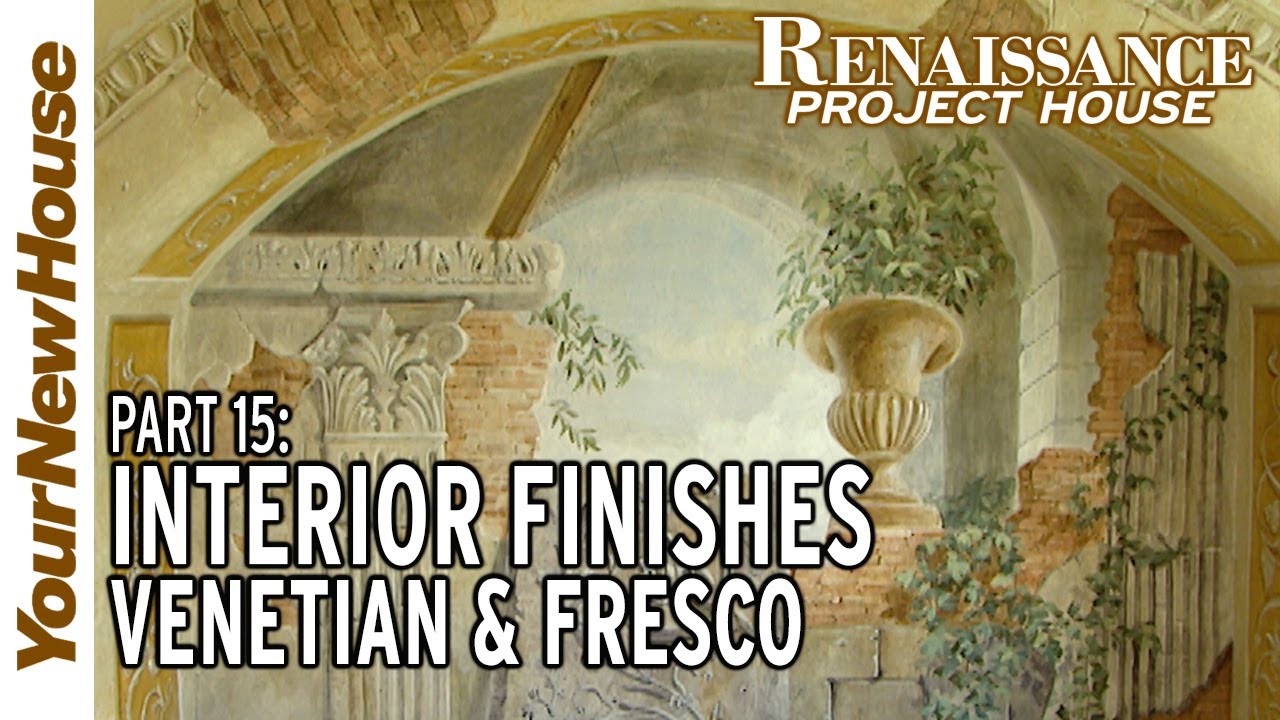This image appears to be an advertisement or thumbnail depicting a painting of an interior space styled in a Renaissance and Venetian fresco theme. The artwork showcases a close-up of an arched interior adorned with large planters, columns, and brick elements. Text is strategically overlaid on the image: on the left side, reading vertically from bottom to top in brown font, it says "Your New House" with capitalized 'Y' and 'H'; at the top right in white font with an orange or rust outline, it reads "Renaissance Project House"; and at the bottom left, it declares "Part 15 Interior Finishes Venetian and Fresco" in white text with a black outline. The interior depicted combines classical Greek and Roman architectural elements with an abstract quality, featuring exposed brick, etched gold or yellowish paneling, and lush plant life climbing the walls and contained in vases. The main visual is a blend of classical architecture and artistic abstraction, reflecting detailed and elegant design elements consistent with Renaissance aesthetics.